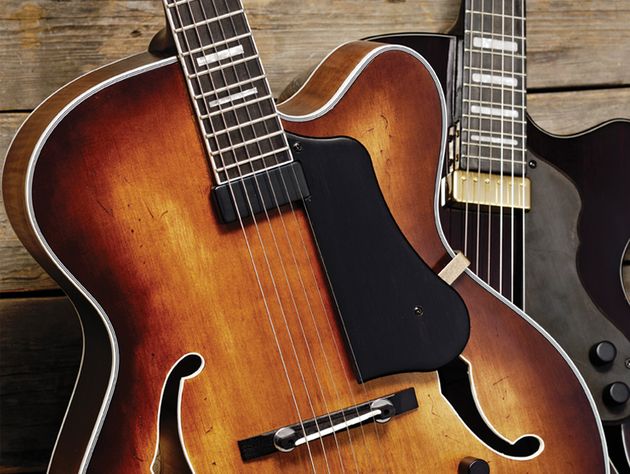The image depicts a medium close-up shot of two guitars, leaning against a wooden wall made of dark, horizontal planks. The foreground guitar is an acoustic guitar with a well-worn look, showcasing a deep brown to light amber sunburst gradient on its body with white-bordered edges. Unlike typical acoustic guitars with a single circular sound hole, this guitar features two distinct, stylish cutout holes. The visible part spans from about a foot above the bottom of the guitar to roughly midway up its neck, revealing its silver strings.

Behind the acoustic guitar, partially obscured, is a sleek black electric guitar. The black guitar, characterized by its glossy plastic finish, is positioned at a slight angle to the right, almost parallel to the acoustic guitar's angle. Both guitars are similarly angled—one slightly left and the other slightly right—giving the impression of a balanced but dynamic composition.